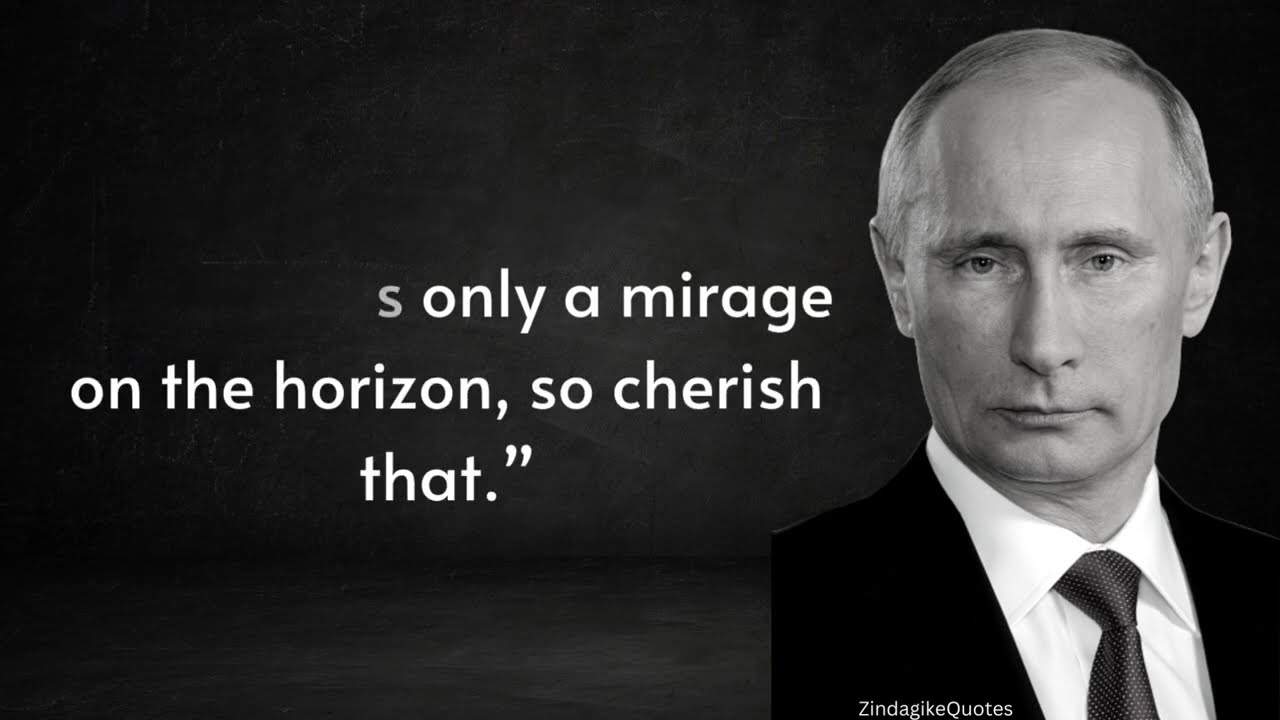This black-and-white image features a serious portrait of Vladimir Putin, the President of Russia, positioned on the right side. Putin is depicted wearing a black suit, a white button-up shirt, and a dark tie adorned with small white dots. His expression is somber, with no smile, and his short hair, large nose, and small eyebrows further define his features, although the color of his eyes is indiscernible due to the monochrome palette. The background of the image resembles an aged, dark slate gray wall and floor, giving the scene a worn, almost dusty appearance. On the left side of the image, white text appears, though the first part is partially erased, leaving only the letter "S" visible. The remaining text reads, "S, only a mirage on the horizon. So cherish that." This quote is accompanied by a notation at the bottom right that says "Zengaki" in small white text.